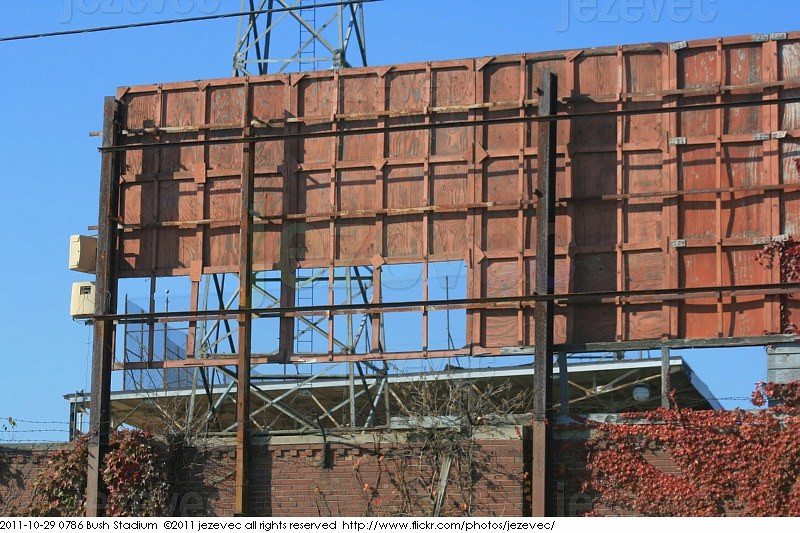In this detailed photograph, we observe the reverse side of a billboard, showcasing the intricate metal framework and poles essential for its support. The structure is affixed to a brick facade, presumably part of a larger building. Lower in the image, a date and title are visible, reading "2011/10/29 0786," followed by the label "Bush Stadium." Additionally, it mentions "Flickr.com photo Zizovec," indicating the source of the image.

Bush Stadium, home to the St. Louis Cardinals baseball team in Missouri, suggests that this billboard is installed on, or near, the stadium's walls. The predominant colors are shades of brown—primarily from the metal components and the brick background—along with the darker tones of the metal poles. The image captures the often-unseen structural side of an advertising billboard in a sports venue setting.